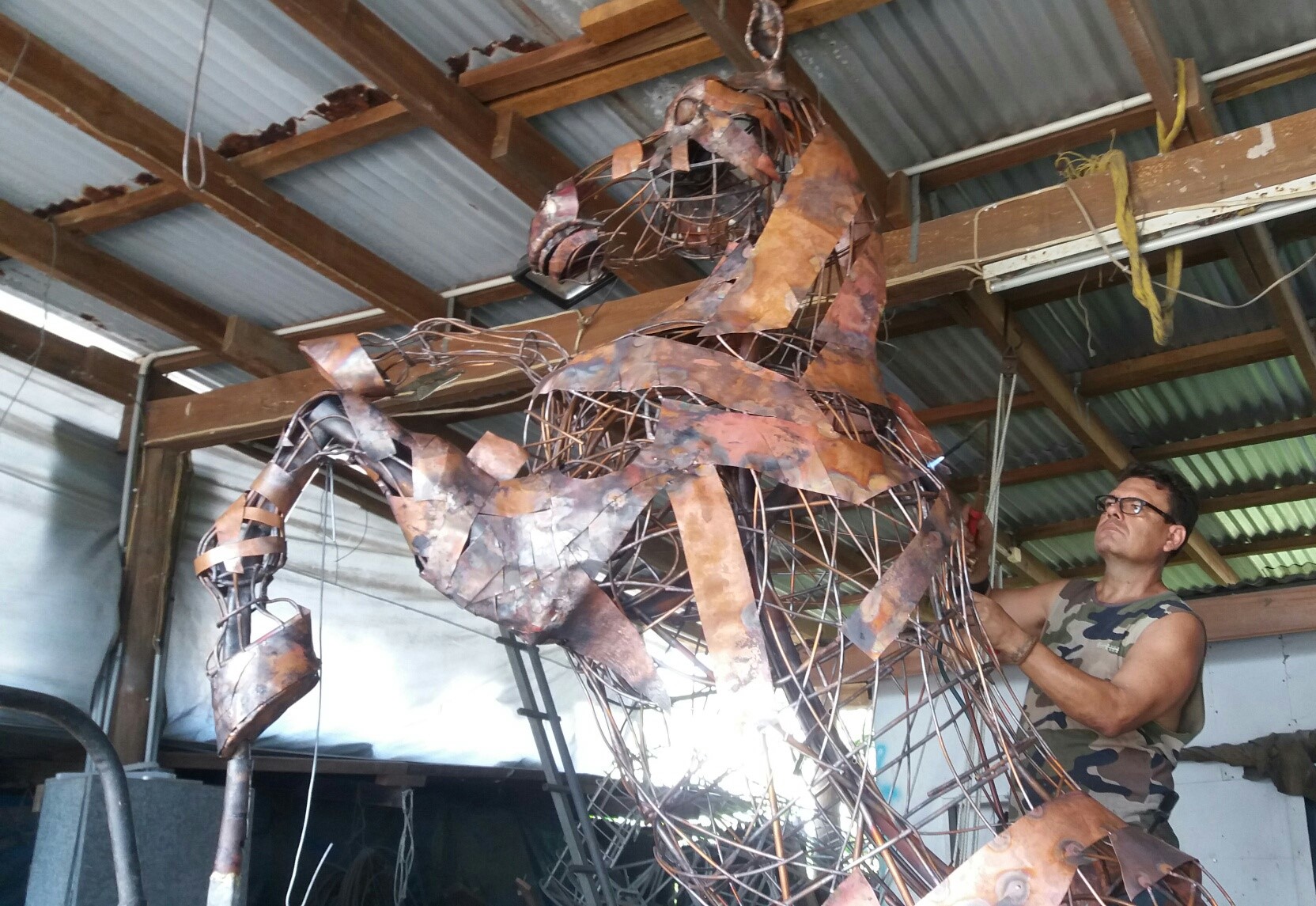In a factory-like setting with white sheet metal roofing supported by wooden planks and walls partially covered with white tarp, a man in his 40s meticulously works on a metal sculpture of a rearing horse. The artist, distinguished by his short black hair, black-rimmed glasses, and a sleeveless green camouflage shirt, is captured on the right side of the frame as he holds metal rods. The horse, currently a detailed wire frame portraying realistic motion, has its neck and head adorned with strips of copper metal, including intricate details such as the eyes and mouth. The workspace also features a visible black element running along and under a shelf area on the left-hand side.